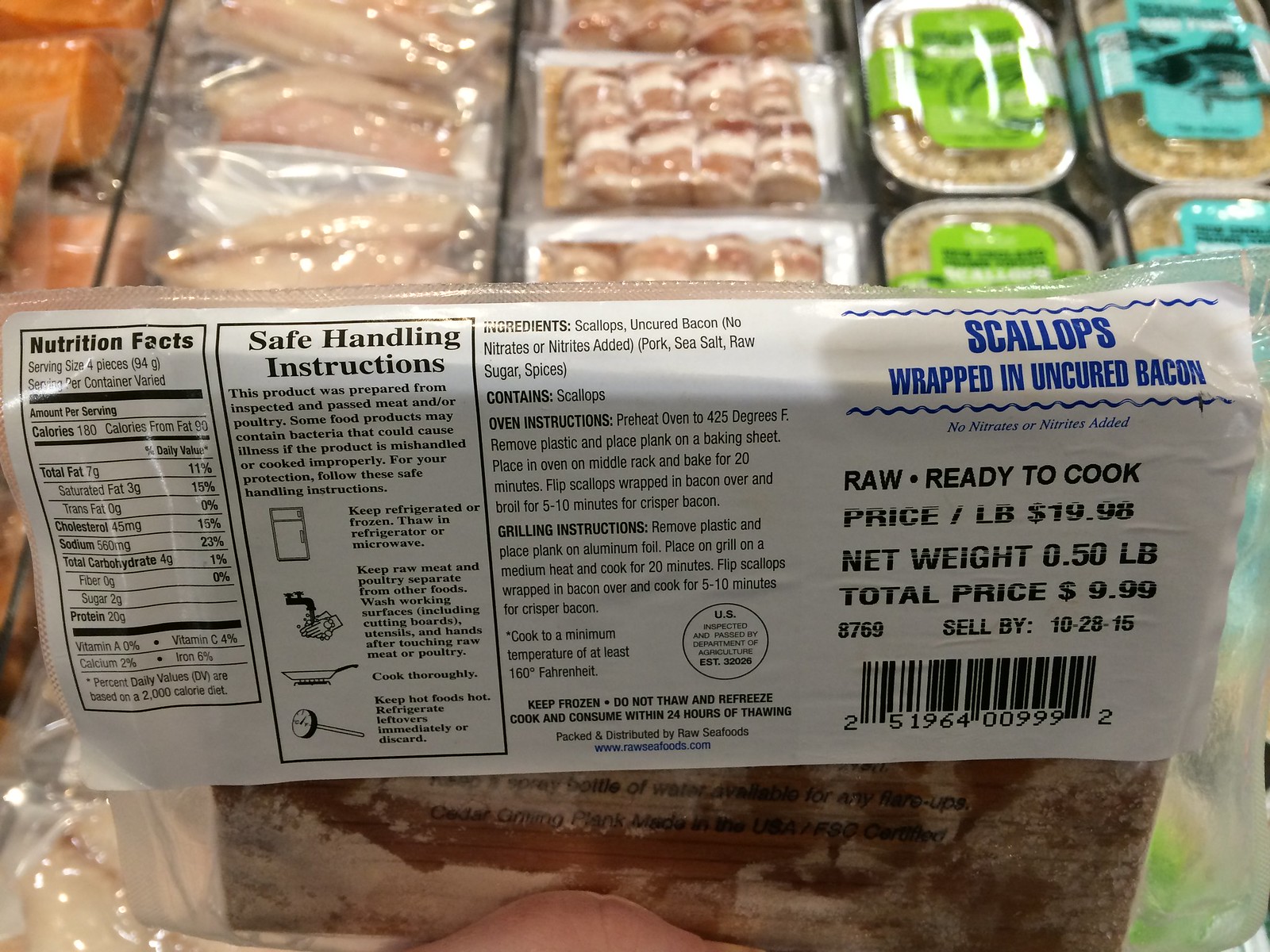This close-up image taken in a butcher shop or grocery store showcases a freezer container filled with various plastic-wrapped pieces of fish. In the foreground, a prominently displayed package of scallops wrapped in uncured bacon steals the focus. The package, supported by a stand, reveals detailed black writing on a white label, including safe handling instructions, nutritional facts, ingredients, and a sell-by date of October 28, 2016. The label features blue writing highlighting "scallops wrapped in uncured bacon" and specifies that they are "raw and ready to cook." The price per pound is $19.98, with a net weight of 0.5 pounds and a total price of $9.99. To the left of this package, there are orangish pieces of fish, white fillets, and other packages potentially containing scallops, all organized in plastic packets and cartons, some in silver trays. In the background, additional bays separated by glass dividers hold a variety of other food items, maintaining the overall setting of a well-stocked and meticulously organized grocery freezer section.